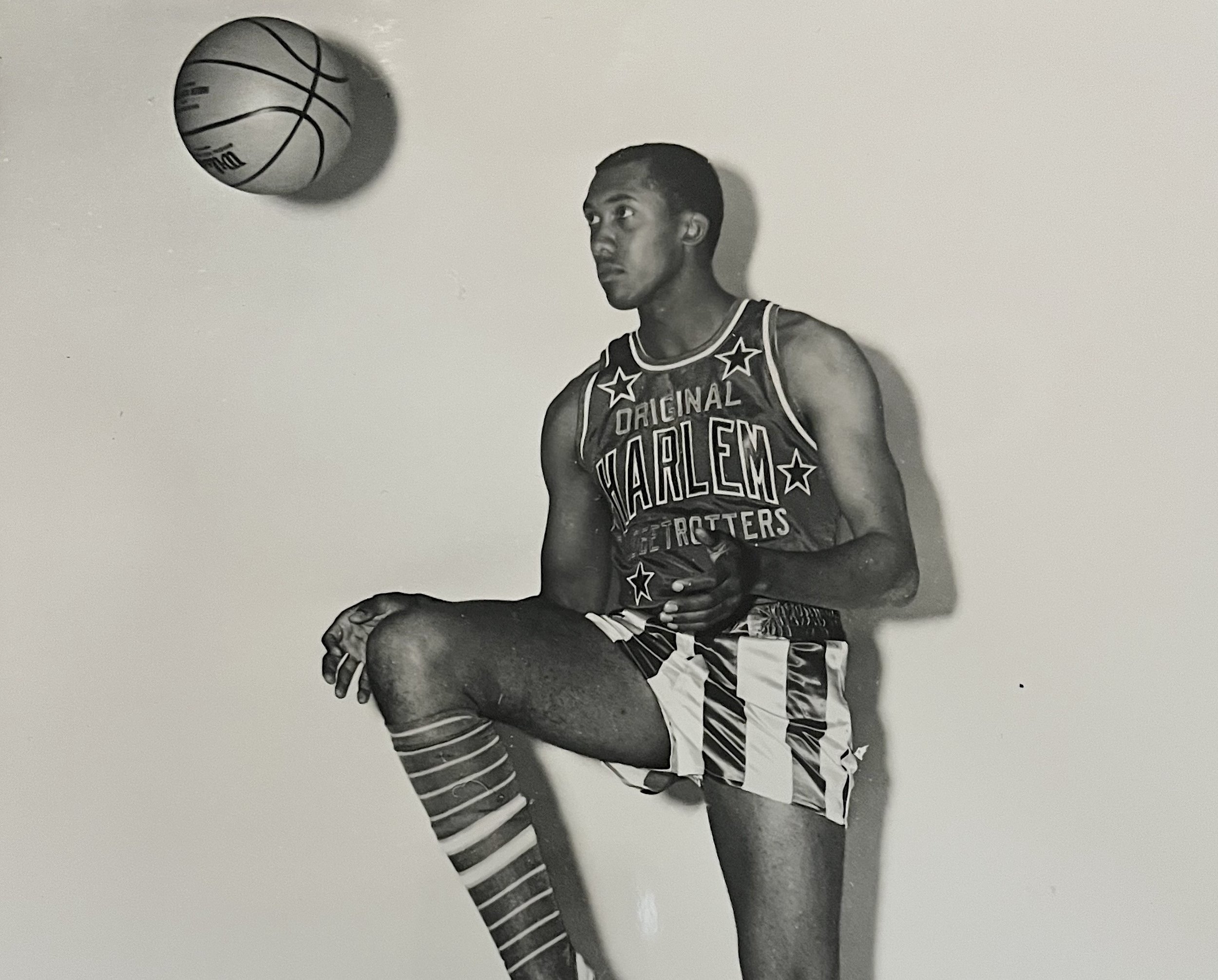This black-and-white photograph captures an African American athlete, a basketball player from the original Harlem Globetrotters, leaning against a white wall with distinctive shadows cast behind him. The focus is on his intricate pose, with his right knee raised to hip height, seemingly juggling a basketball in the air towards the upper left corner, his eyes intently following its trajectory. He is clad in the iconic Harlem Globetrotters uniform: a dark-colored jersey adorned with stars and the text "Original Harlem Globetrotters," complemented by vertical striped shorts with a black waistband, and knee-high socks featuring horizontal stripes. The light, coming from straight ahead, accentuates the scene, emphasizing the nostalgic, old-school essence of this meticulously posed image.